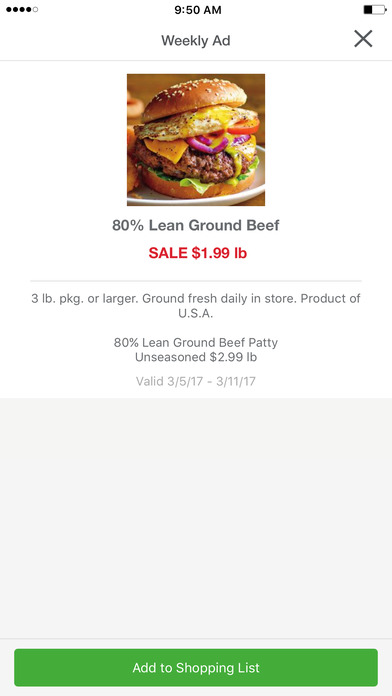In the image, there is an advertisement banner showcasing a detailed list of food items and promotional offers. At the top, there are numbered sections "1, 2, 3, 4" followed by a category labeled "Tots." The highlighted item is priced at 950 meters and marked "Knot." Nearby, the phrase "Battery, Weekly Head, Eggs, Easy Burger" stands out, suggesting a focus on food. 

The centerpiece features "12 Buns," with a specific callout for the "Bun of the Month," which includes ingredients like meat, tomato, eggs, cheese, and red onion. The burger is elaborated to be made from 80% lean ground beef, currently on sale for $1.99 per pound. The dates "3/5/17 - 3/11/17" likely indicate the duration of the sale or promotion.

On the right, there’s a grey square and below it, a green rectangle prominently labeled "Add to Shopping List." This structured layout and these vibrant colors give a clear call-to-action, enhancing the visual appeal as a background image.